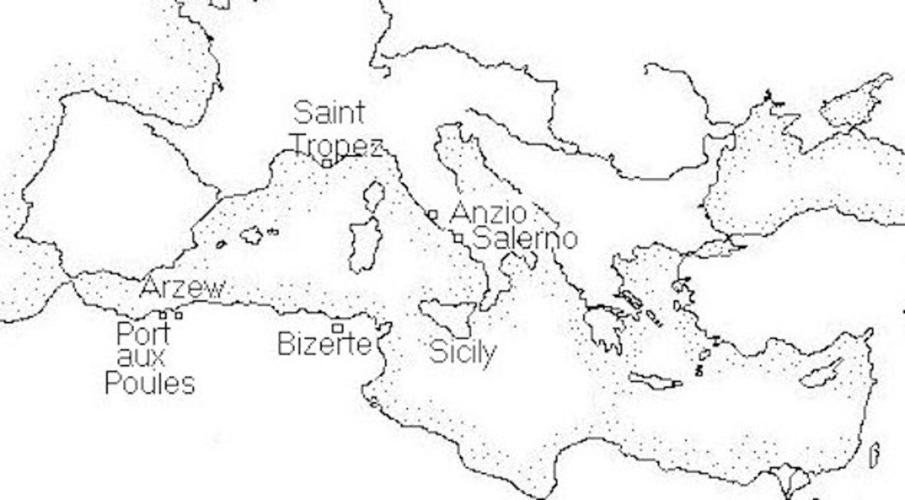The image is a basic black and white drawing of a map depicting parts of Europe, specifically the regions around France and Italy. It includes labeled cities such as Saint-Tropez, Anzio, Salerno, Sicily, Bizerte, Arzu, and Port Auxpolis. The landmass is distinguished by an inner border decorated with numerous small black dots, adding a hatch-like fill inside the outlined countries. The map is devoid of any other detailed elements such as keys or color, focusing solely on the geographic outlines and the names of the cities.